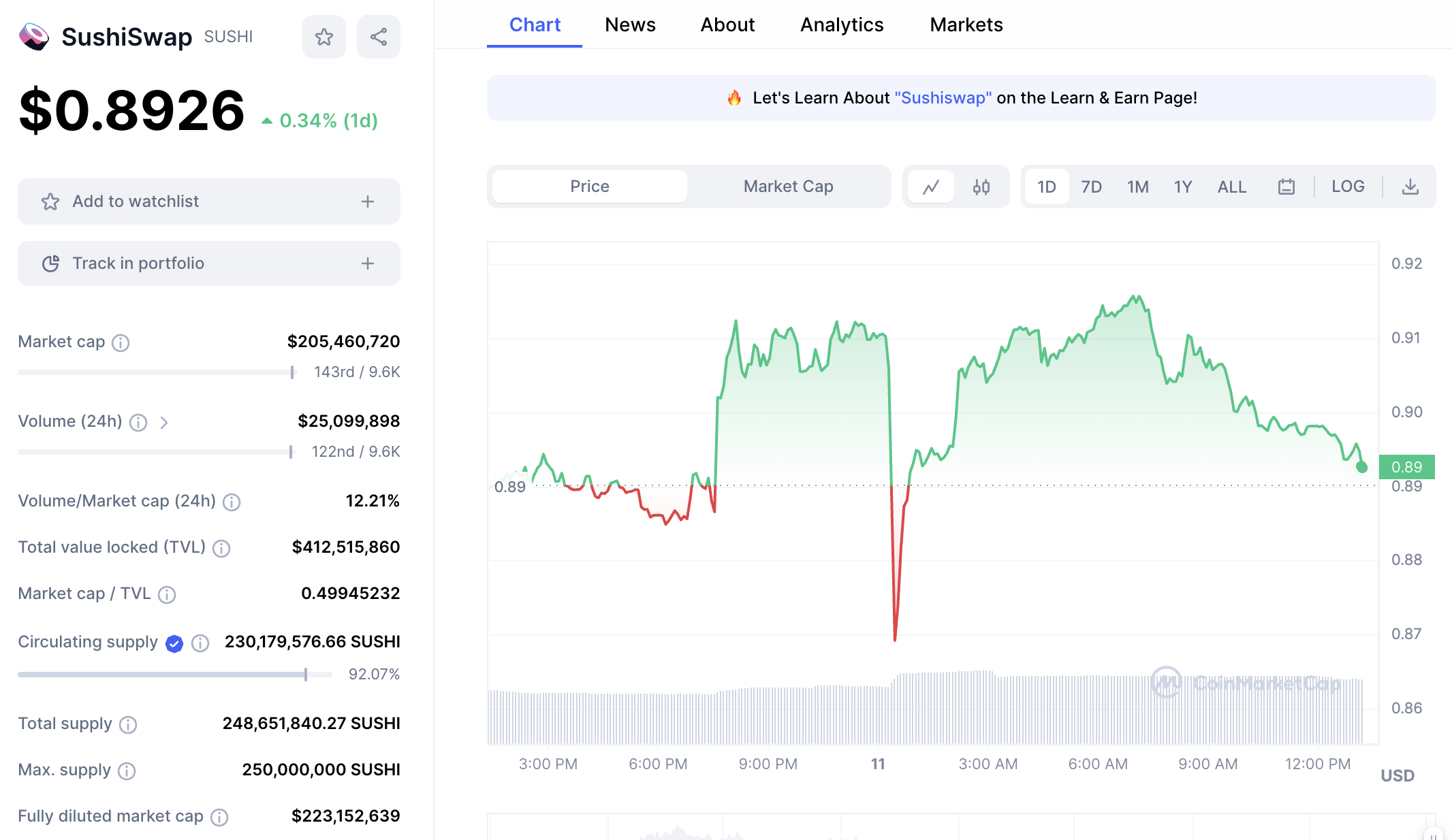The rectangular image, oriented horizontally, features a clean white background. On the left-hand side, taking up roughly one-quarter to one-third of the image, there is a vertically aligned section labeled "SushiSwap." Next to this label, there is an icon of a sushi roll, followed by a star icon and a share button. Below these elements, bold black text displays "$0.8926," indicating the current value of the asset. Additionally, a smaller text below it notes that this value is up by 0.34% for the day. 

Further down in the same column, there are options for "Add to Watch List" and "Track in Portfolio," suggesting that the image might be from a financial or investment platform. Key financial metrics are listed, including "Market Cap" at $205,467.20, and "Volume (24h)" at $25,000,099.99. Other financial details such as Volume Cap, Total Value Locked, Market Cap, Circulating Supply, Total Max Supply, and Fully Diluted Market Cap are also mentioned but not fully detailed in the description.

On the right-hand side, which occupies the remaining portion of the image, there's a horizontal navigation menu at the top. The menu items are "Chart," "News," "About," "Analytics," and "Markets." The "Chart" option is currently selected, indicated by its blue color and an underline, while the other menu items are in black. This section likely displays the visual chart and data related to the SushiSwap asset.